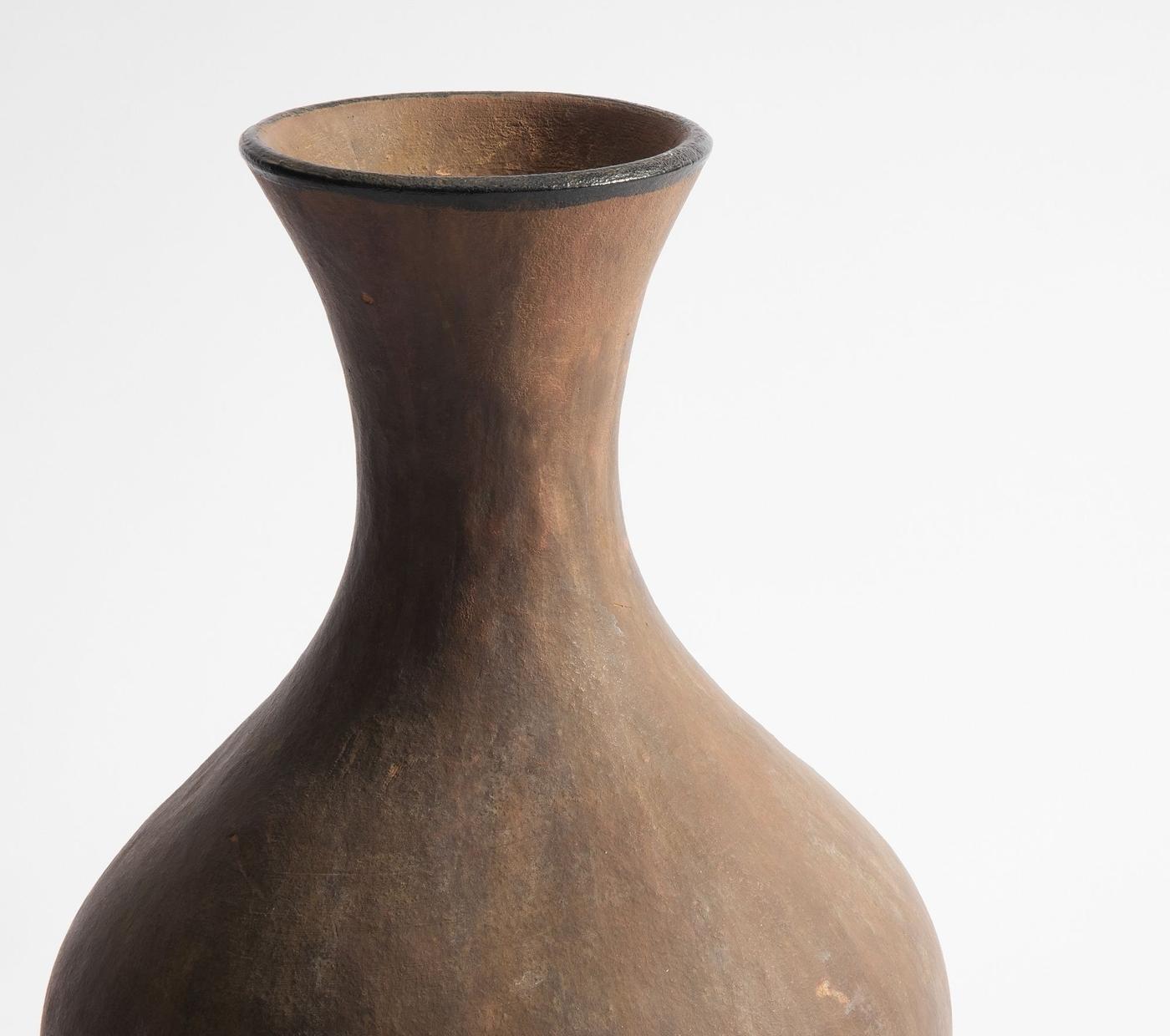This photograph showcases a close-up view of the upper portion of a vase against a white background. The vase, which is made of dark brown clay, features a smooth, matte finish without any text, design, pattern, or engraving. The neck of the vase is narrow and curves inward before flaring out at the shoulders. The rim at the top is distinguished by a black ring, contrasting with the brown body. The image only captures the vase from the shoulders up, leaving the bottom unseen, and emphasizes the natural, minimalist aesthetic of the clay object.